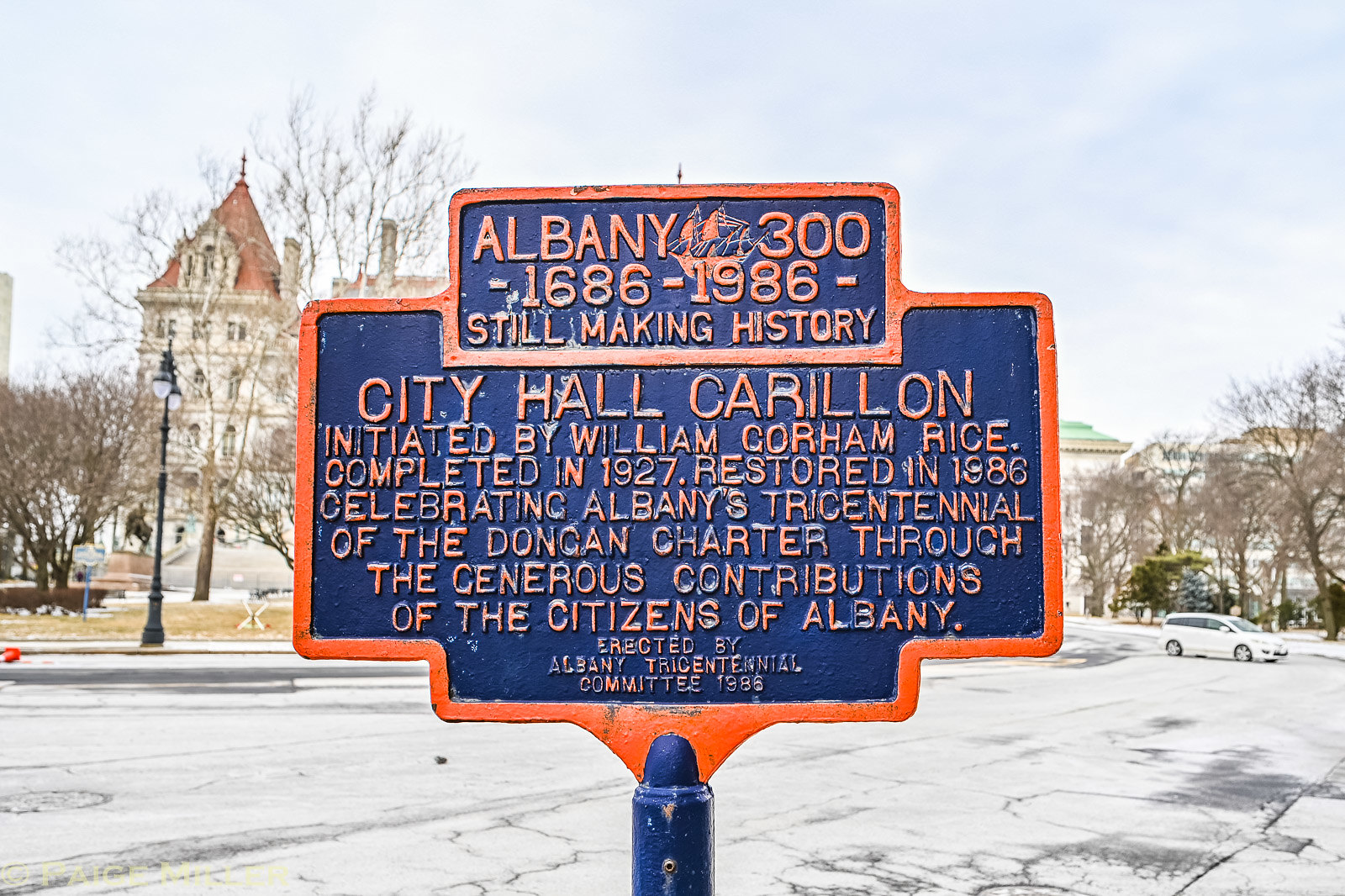A detailed photograph captures a commemorative painted metal street sign with a medium blue background and a striking orange border. The text on the sign, also in orange, reads: "Albany 300, 1686-1986, still making history. City Hall, Carillon, initiated by William Gorham Rice, completed in 1927, restored in 1986, celebrating Albany's tricentennial of the Dongan Charter through the generous contributions of the citizens of Albany, erected by Albany Tricentennial Committee, 1986." The top of the sign pole is visible, rooted firmly in a setting with a parking lot and a broad street behind it. The background also features a notable building on the right, distinguished by its pointed red roof and a black street light in front of it. To the right of the sign, a white car is parked, partially obscured by trees and bushes. The sky overhead is mostly cloudy with patches of light blue, adding to the vivid scene.